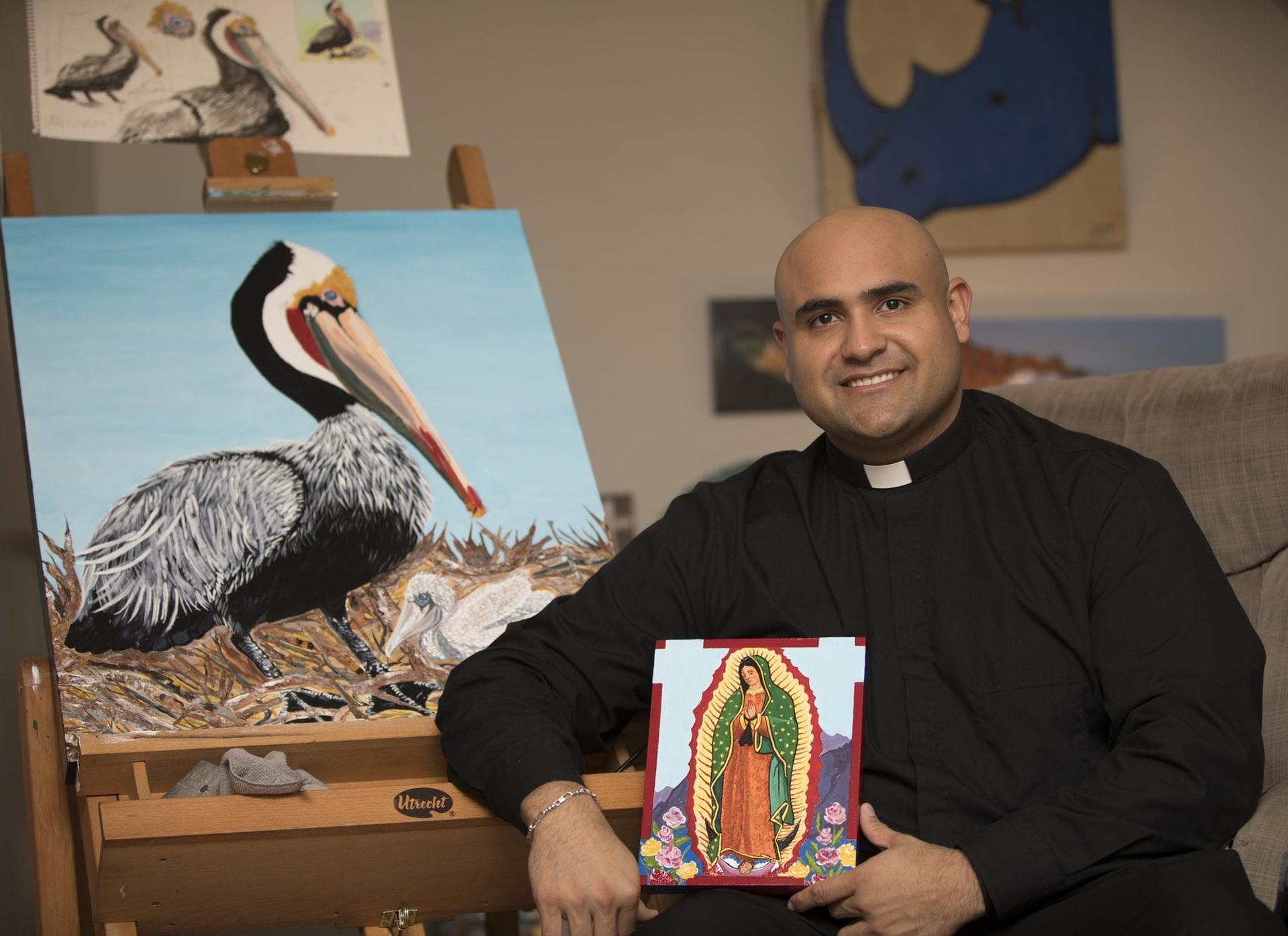In this landscape-oriented photograph, a smiling priest with medium brown skin and no hair gazes directly at the camera. He is dressed in a traditional black cleric's outfit with a white collar. His right arm rests on an easel marked with "Utrecht" while his left hand holds a vibrant painting of a woman in an orange dress and green shawl, surrounded by flowers on a red background, resembling a female religious icon. The easel also features a detailed painting of a gray and black duck with colorful markings—white, yellow, red, and green—on its face and beak, potentially confused with a pelican in other depictions. Above this, several sketches show the bird in various poses. In the background, slightly out of focus, is a striking painting of a blue rhinoceros on a tan canvas. Additionally, the priest sports a silver bracelet on his right wrist, adding a touch of personal style to his otherwise traditional appearance.